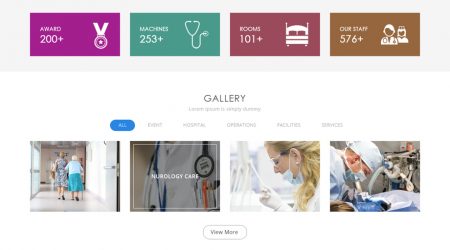The image is a screenshot from a website with a clean and streamlined design. The top portion features a gray background, which includes four small, colored rectangles, each representing different categories with corresponding icons and statistics. 

1. The first rectangle is plum-colored and displays the text "AWARDS 200+" alongside an icon of a medal, typically worn around the neck.
2. The second rectangle is jade-colored, displaying "MACHINES 253+" with an icon of a stethoscope.
3. The third rectangle is muted burgundy and reads "ROOMS 101+" in capital letters, accompanied by an icon of a bed.
4. The fourth rectangle is light brown, showing "OUR STAFF 576+" with icons representing a doctor and a nurse.

Below this section, the background turns white, with the word "GALLERY" in bold, capital letters in the center. Beneath "GALLERY," there is a subtitle in faint text that reads "All event hospital operations facilities and services."

Further down the page, there are four square images arranged side by side, likely showcasing various aspects of the hospital's operations and facilities. At the very bottom, there is a light gray tab that says "View More," prompting users to explore additional content.